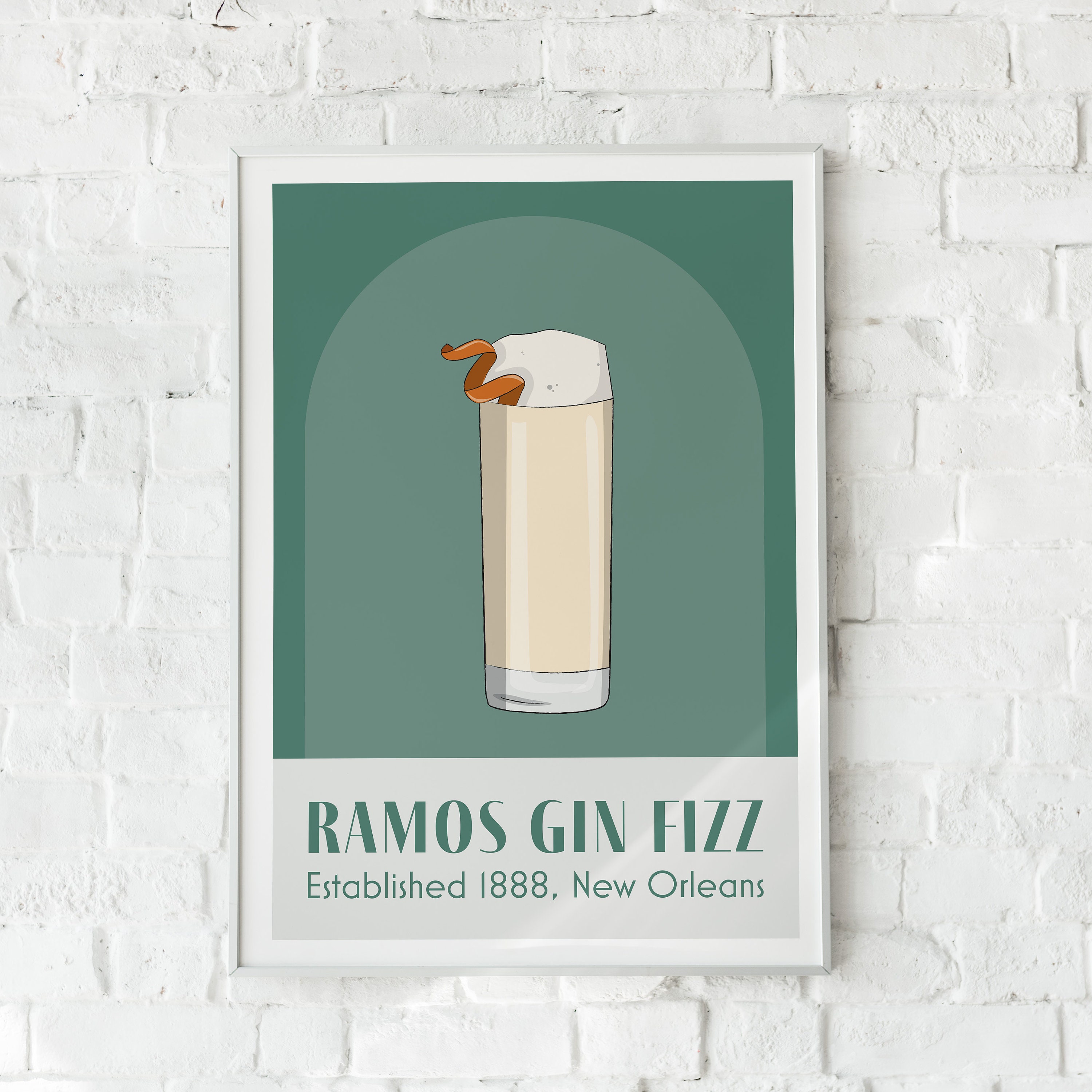This detailed image depicts framed wall art mounted on a white-painted brick wall. The art itself is an advertisement-style drawing enclosed in a thin white rectangular frame. The focal point of the artwork is a tall, slender highball glass filled with a tan-colored Ramos Gin Fizz, complete with a generous topping of white foam. A curly piece of orange rind protrudes elegantly from the foam. The drink is set against a dark green background featuring a light green arch shape in the middle. Beneath the glass, text in capital letters reads "Ramos Gin Fizz," with the subtitle "Established 1888, New Orleans."